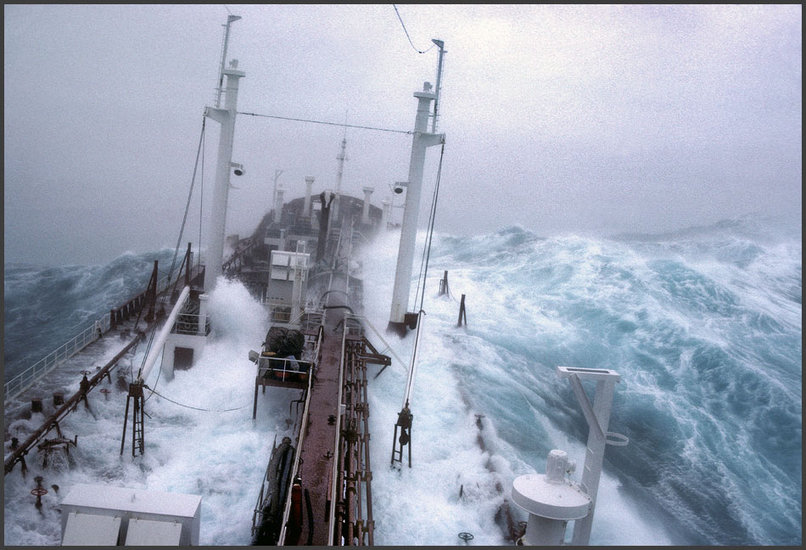The image depicts a massive ship battling against the ferocious waves in the middle of the ocean. Positioned prominently on the left side of the frame, the ship appears to be nearly submerged by a series of immense, bluish-teal waves with frothy white caps. The relentless waves have overflowed onto the deck, and the vessel seems to be struggling to stay afloat under the sheer volume of water cascading over it. 

Amidst this tumultuous setting, large white poles and a sturdy beam or walkway stretch across the ship's expanse, hinting at an underground section where the crew might be sheltered. Despite this, the ship's dire state suggests it's on the brink of sinking. 

The sky above is a grim gray, with a slight white haze in the middle where the sun attempts to pierce through the clouds. The image, likely captured from an aerial perspective, hints at a high degree of noise and possible digital artifacts, with some elements appearing unnaturally smooth, leading to speculation that it might be AI-generated. A black border frames the image, adding to the overall impression of a harrowing sea storm engulfing the large vessel.